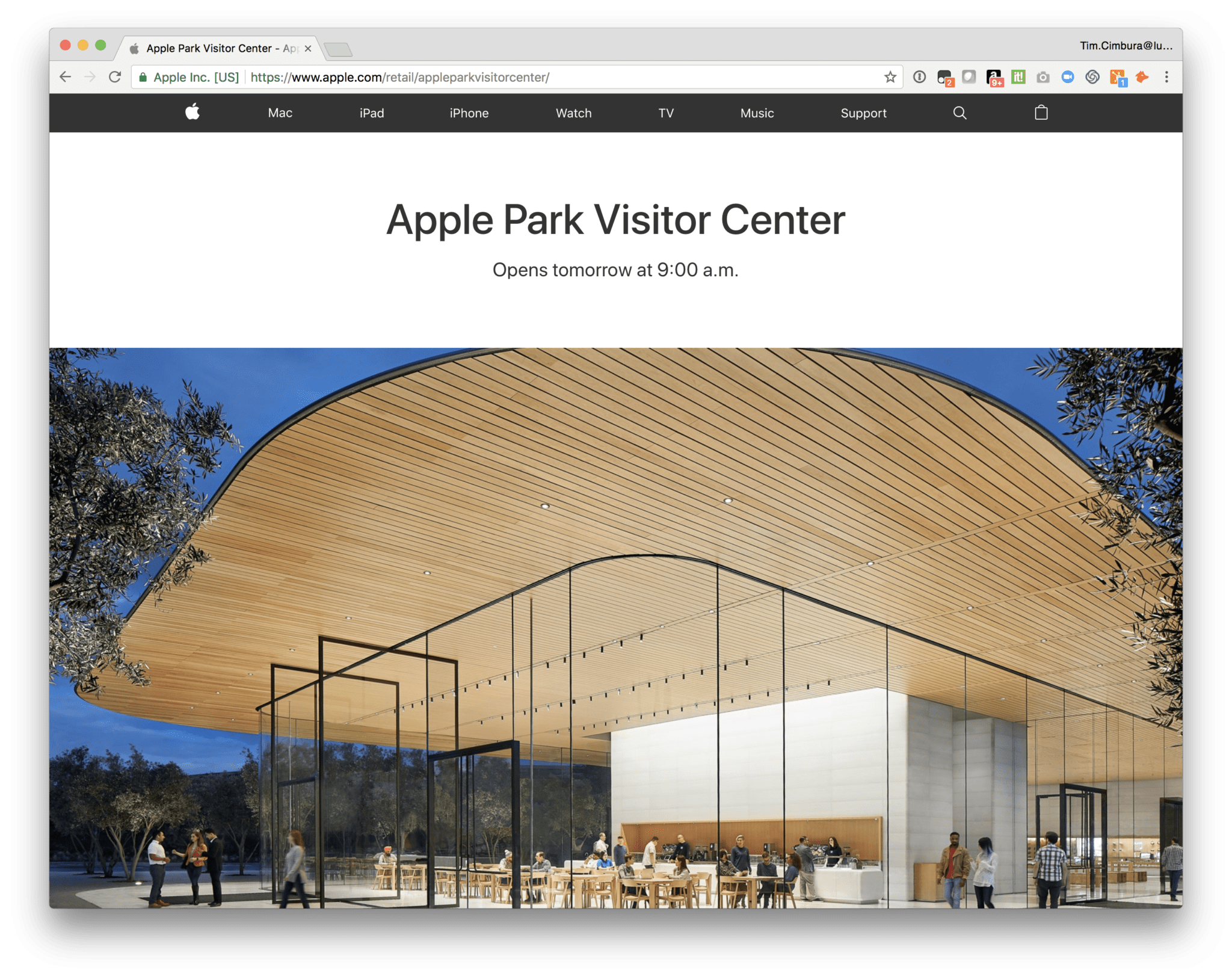A screenshot captures a webpage being viewed in a browser. The browser's top section is gray, featuring three horizontal dots in red, yellow, and green. Adjacent to these, the current tab displays the Apple logo followed by the text "Apple Park Visitor Center." In the upper right-hand corner of the browser, an email address begins with "tim.klimvira.at," but is cut off in the image.

Beneath the tab area, browser navigation options are visible, including back and forward arrows, a refresh button, and the URL "https://www.apple.com/retail/apple-park-visitor-center," indicating the page's secure connection to Apple's official website. A favorites button and several extension icons in black, green, and orange hues are also present, though unidentifiable.

The web page itself features a black header bar with the Apple logo and links to various sections: Mac, iPad, iPhone, Watch, TV, Music, Support, Search, and a shopping bag icon. Below this, a white banner announces "Apple Park Visitor Center opens tomorrow at 9 a.m."

The main content of the webpage is an image of the Apple Park Visitor Center, showcasing its architectural details. The Visitor Center has a brown wood panel design beneath scaffolding, glass doorways, oak-colored tables, and a bar area, all contributing to its modern and inviting aesthetic.